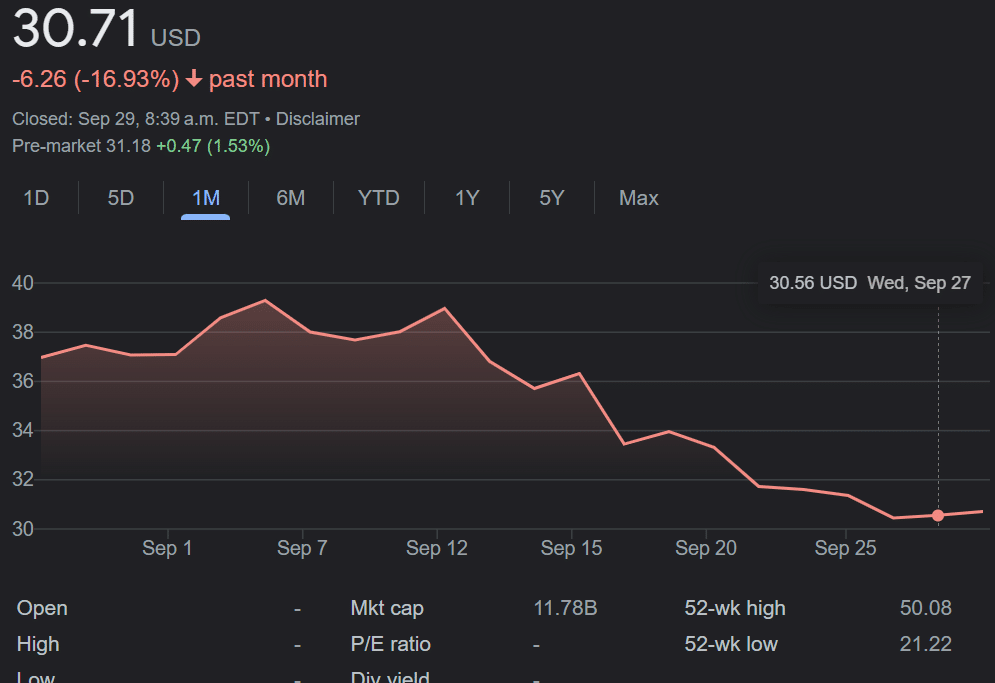The image displays a financial chart with a black background. In the top left corner, the current price is shown as "30.71 USD." Directly below that, the date is displayed in grey text. Along the bottom section of the image, financial changes for the past month are noted with details in red: a decrease of "6.26" units or "16.93%" is indicated by a downward arrow followed by the phrase "past month."

Additionally, text at the bottom includes the status "Closed September 29, 8:89 a.m. EDT," along with a disclaimer about pre-market changes. The pre-market value is listed as "31.18," reflecting a positive change of "+0.47 (1.53%)," with both the increase "0.47" and percentage "1.53%" highlighted in green.

In the next section, a blue-highlighted timeframe selector indicates "one month" as the current view. The options available are: one day, five days, one month, six months, one year, five years, and max.

Beneath this, a red line graph provides a visual representation of the market's progress over the selected month. The y-axis is graduated in increments from 30 to 40, and the x-axis ranges from September 1 to September 25. Key metrics including "Open," "High," "Low," "Market Cap," "P/E Ratio," "Dividend Yield," "52-Week High," and "52-Week Low" are listed. Specifically noted are the market cap of "11.78B," a 52-week high of "50.08," and a 52-week low of "21.22."